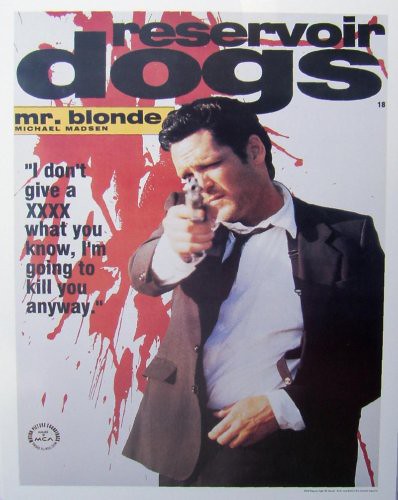This magazine cover features a striking advertisement for the movie "Reservoir Dogs." The title "Reservoir Dogs" is prominently displayed at the top in bold black letters. Below the title, there is a vivid yellow strip extending from the top of the man's head to the left side of the cover, labeled "Mr. Blonde Michael Madsen." Beneath this strip, a chilling quote reads, "I don't give a XXXX what you know, I'm going to kill you anyway," enclosed in quotation marks.

Dominating the cover is a photograph of Michael Madsen, who is depicted as Mr. Blonde. He is a Caucasian man in his 40s to early 50s, wearing a black suit with a white collared shirt and a black tie. He has black hair and his pale skin contrasts sharply with the colors around him. Madsen's character is seen pointing a gun directly at the viewer, adding an intense and confrontational element to the image. The background features a dramatic red splatter, resembling either blood or paint, set against a white backdrop, enhancing the overall intensity of the cover.